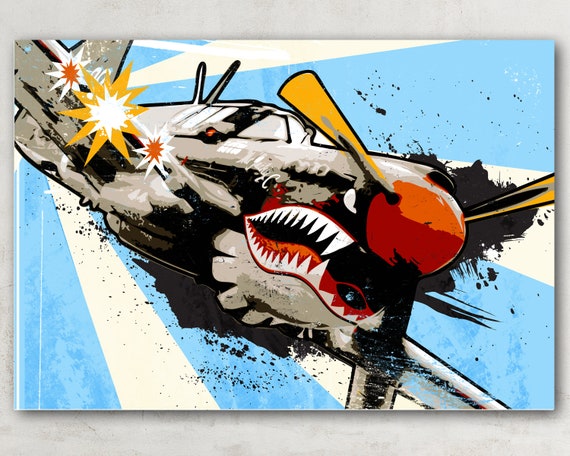The image depicts an abstract, colorful painting on a gray background, featuring a stylized World War II era fighter plane. The painting is rectangular and wider than it is tall, with a background of sky blue and cream-colored stripes. The plane, rendered in a cartoonish and anthropomorphic manner, has a vivid red nose and yellow propellers, tilted at a 45-degree angle, suggesting high speed. Its body is primarily gray with black and green shades, adorned with a menacing shark face—a red mouth brimming with sharp white teeth, and slanted white eyes conveying anger. White streaks and explosive flashes of yellow, white, and red around the wings illustrate the plane engaged in a fierce dogfight, enhancing the dynamic and aggressive feel of the artwork.